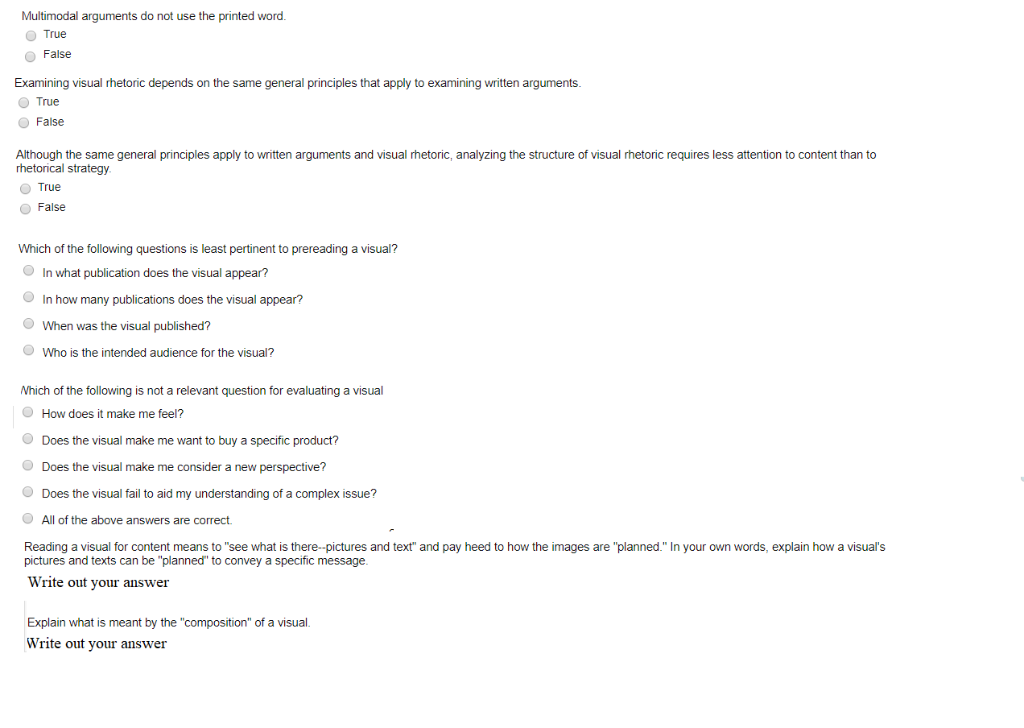The image displays a detailed web page from a website, focusing on visual and written rhetoric analysis. At the top, black text asserts: "Multimodal arguments do not use the printed word," followed by true and false bubbles for user interaction. Below, the text reads: "Examining visual rhetoric depends on the same general principles that apply to examining written arguments," also accompanied by true and false bubbles.

Subsequent text states: "All of the same general principles apply to written arguments and visual rhetoric. Analyzing the structure of visual rhetoric requires less attention to content than to rhetorical strategy," followed by another set of true and false response bubbles.

The next section asks: "Which of the following questions is least pertinent to pre-reading a visual?" Users are presented with multiple choice bubbles, leading to text on the right of each bubble, listed in descending order: "In what publication does the visual appear?", "How many publications does the visual appear?", "What was the visual?", "When was the visual published?", and "Who was the intended audience for the visual?"

Following this, the web page poses: "Which of the following is not a relevant question for evaluating a visual?" The available bubble choices with corresponding text on their right, in descending order, are: "How does it make me feel?", "Does the visual make me want to buy a specific product?", "Does the visual make me consider a new perspective?", and "Does the visual fail to aid my understanding of a complex issue?" The statement concludes with: "All of the above answers are correct."

Further down, the text explains that "Reading a visual for content means to 'see what is there—pictures and text,' and pay heed to how the images are 'planned'." Below this instruction, users are asked: "In your own words, explain how a visual's picture and text can be 'planned' to convey a specific message." An input box is provided for users to write their answers.

The final prompt reads: "Explain what is meant by 'composition' of the visual," followed by another text box for users to provide their written responses.